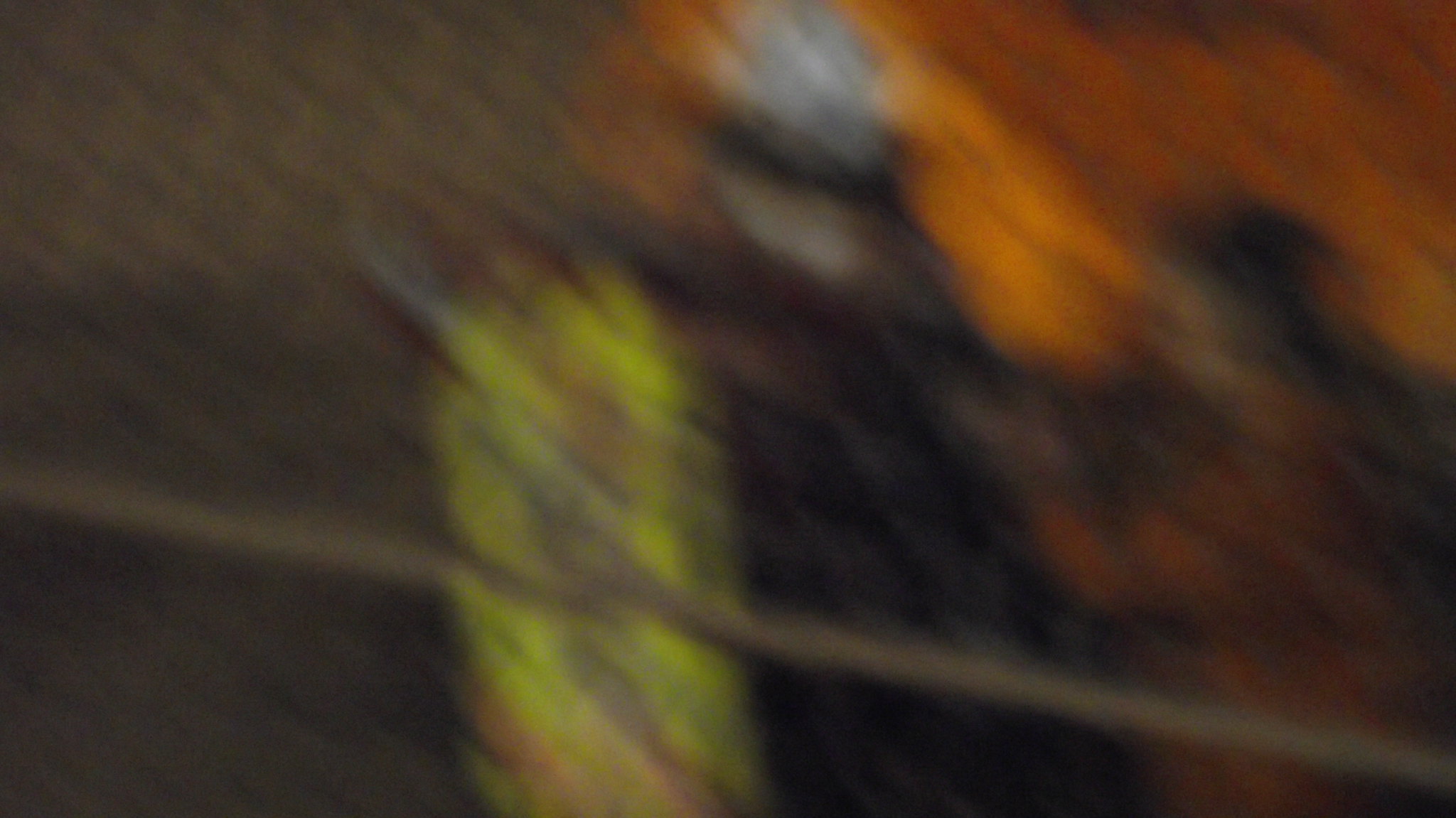The photograph is a color image in landscape orientation that is extremely blurred, making it difficult to discern the specific contents. The entirety of the foreground is covered by a chain-link fence, with a thicker diagonal line from the upper left to the bottom right, likely indicating a reinforced section of the fence. A yellow steel pole, showing signs of rust at its base, is visible slightly left of center, partially obscured by the criss-crossing wires of the fence. In the upper right portion, a vibrant, blurry mass of orange with some darker patches suggests the presence of an animal, possibly an orangutan or tropical bird, though the details are indiscernible. Additionally, there are gray tones and a predominantly dark, nearly black background, contributing to the overall ambiguity of the image.